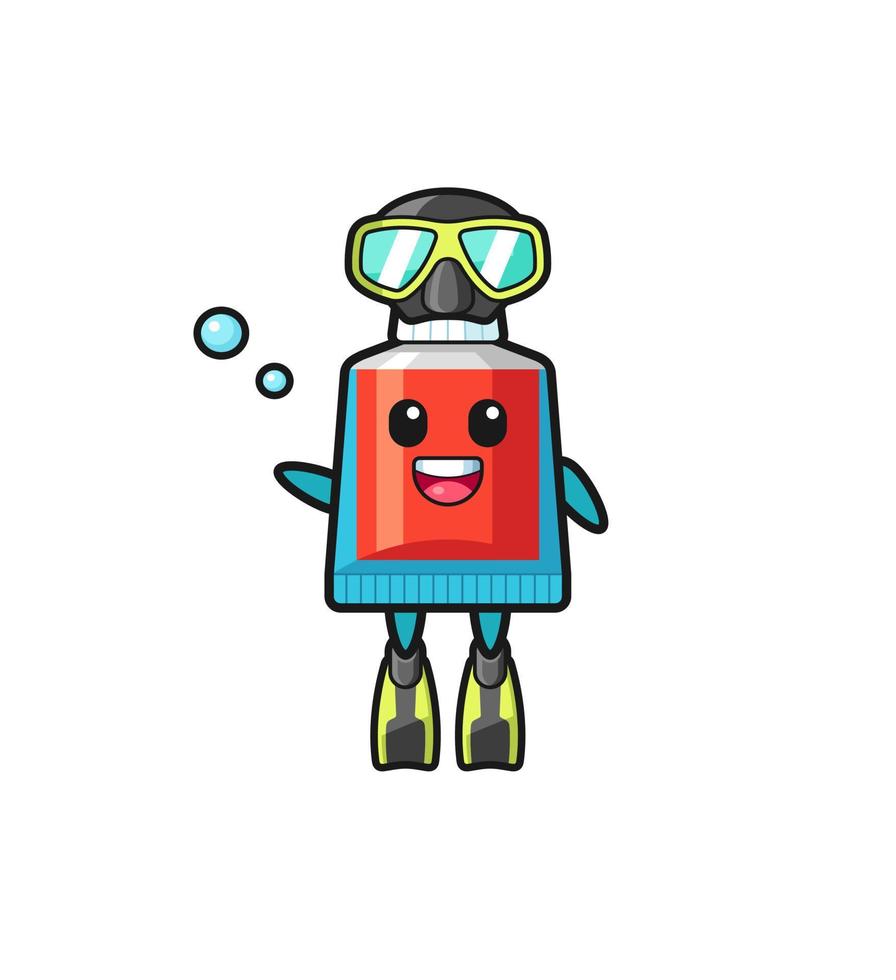The image is a detailed digital illustration of a comic book character resembling a short and stubby tube of toothpaste, though it could also be seen as a bottle of nail polish. The character's body is primarily blue, with a prominent red square in the middle featuring two black eyes and a smiling mouth that shows white teeth and a red tongue. This central red part is equipped with a scuba mask that has a black cap with a nose and yellow goggles with blue interiors and white stripes. It also sports small, flipper-like arms and blue legs that lead down to diving fins, which are a light shade of green with gray streaks and yellow highlights. Additionally, two blue bubbles, outlined in black, emanate from the left, suggesting an underwater setting.